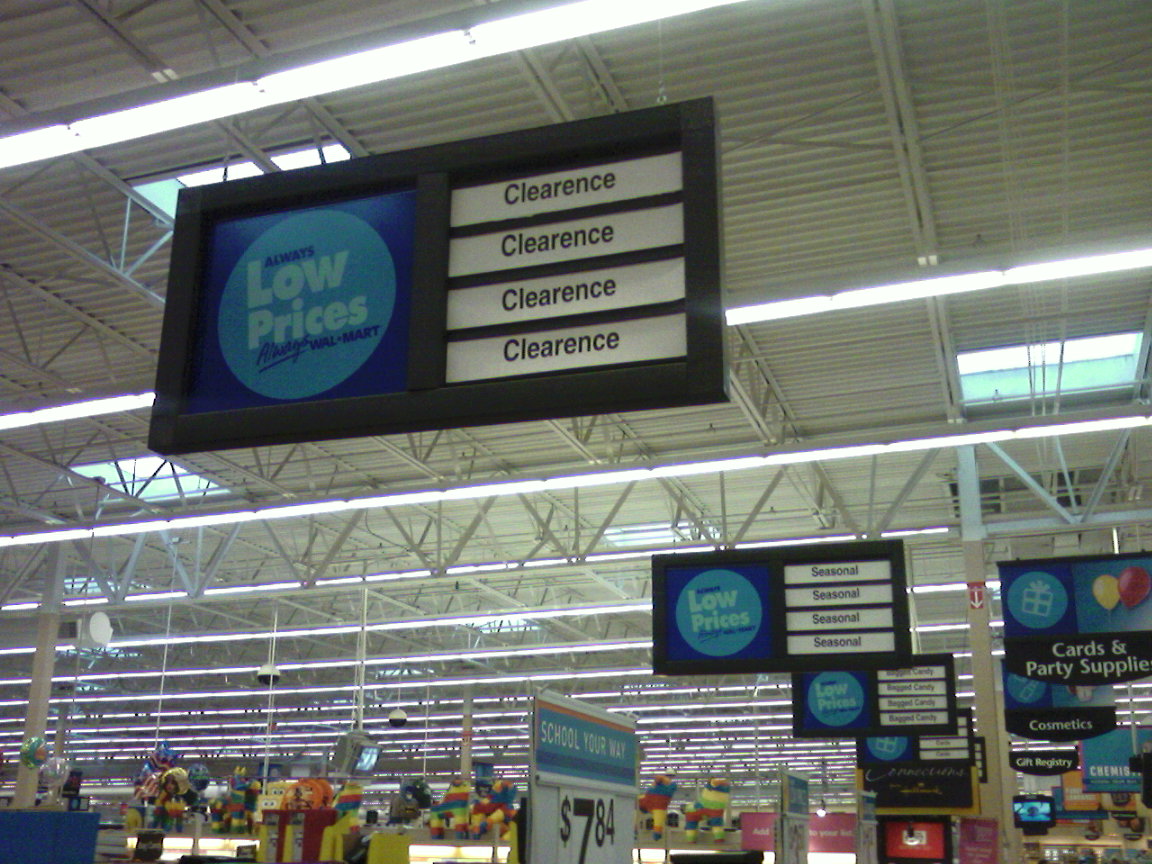This photograph captures the interior of a store that resembles Walmart. Prominently displayed from the ceiling are multiple blue signs featuring a light blue font that reads "Always Low Prices" with "Walmart" written beneath in dark blue. The closest sign to the camera has four white bars with "Clearance" repeated on each. Behind these, additional signs indicating "Seasonal" can be seen, with some reading "Bagged Candy," although they are blurry and difficult to decipher.

In the right section of the image, various store departments are visible, starting with "Cards and Party Supplies," followed by "Cosmetics" and "Gift Registry." Brightly colored piñatas are scattered throughout this area. On the left side of the photograph, a structure that appears to be a self-checkout or scanner of some kind is noticeable. Additional signage includes a promotion for "School Your Way" with a price tag of $7.84. The layout and organization suggest this image was taken near the front of the store.